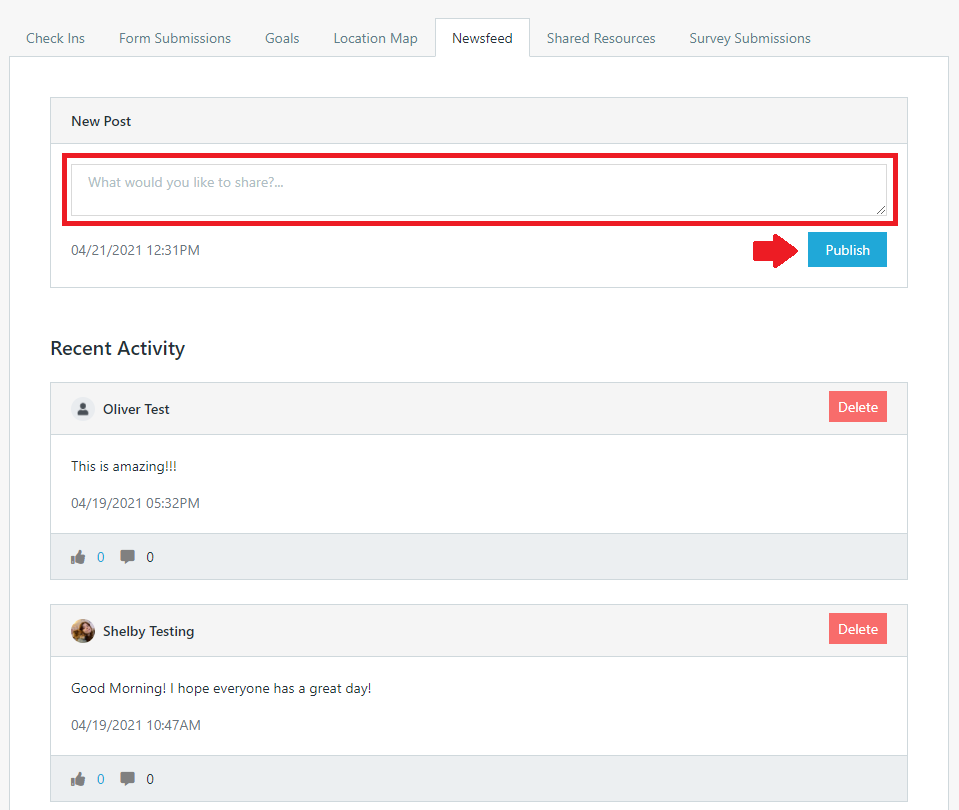The image depicts a vibrant and detailed user interface of an application. Key elements in the interface include various features such as:

1. **Check-ins** and **Surveys Submissions:** Sections likely for user input and feedback.
2. **Foreign Submissions**: Possibly a space for international entries.
3. **Goals, Location Map,** and **New Seed:** Dedicated areas for goal tracking, location visualization, and new entries.
4. **Shared Resources** and **New Post**: Areas for shared materials and new content creation.

Specific UI elements noted are:
- A **Red Border** featuring the prompt "What would you like to share?"
- The identifier **046211 saying 2211** and **231 PM** indicating a specific item and timestamp.
- A significant **Red Arrow** pointing to a "Publish" button against a **Red Background**.
- A **Recent Activity** section mentioning "Oliver Test" and another **Red Square** labeled "Delete."
- An enthusiastic comment, "This is Amazing!"
- Other activities from the user labeled **04619 saying 221**, noting two different times: **532 PM** and **1047 AM**.

Engagement elements include:
- **Thumbs Up** icons next to content confirming user approval or likes.
- **Shelby Testing** noted possibly as a user name or test phase.
- A **Rectangle** and **Circle** both labeled "Delete," indicating multiple UI options for deletion.
- A cheerful greeting: "Good Morning, I hope everyone has a great day."

The interface displays clear, differentiated **White Background Windows** and contains **three distinct rectangular tabs** for navigation or displaying various sections of the application.